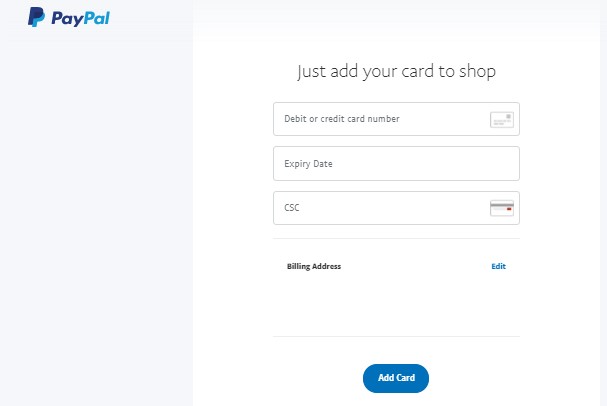This screenshot captures the "Add Your Card to Shop" interface on the PayPal website. The left third of the screen is shaded in light gray and features the PayPal logo and the word "PayPal" at the top. The remaining space on this section is blank. 

On the right side, occupying the main portion of the screen, is a large white background, creating a clean and uncluttered look. At the top, the header reads "Add Your Card to Shop." Below the header are three input fields displayed as rectangles. 

The first rectangle prompts the user to enter their "Debit or Credit Card Number," accompanied by a grey clipart icon of a credit card. Directly below, the second rectangle is for inputting the "Expiry Date," positioned towards the left side of the box. The third and final rectangle asks for the "CSC" (Card Security Code), highlighted with an illustrative icon showing a credit card's back side. The icon features a red section where the CSC number would typically be found, along with a horizontal line representing the card's magnetic strip.

Under these input fields is a gray dividing line followed by the bolded text "Billing Address" and a blue "Edit" link for making changes to the billing address. Further down, after another gray dividing line, is a blue action button labeled "Add Card" in white text, notable for its rounded corners.

The entire page design is minimalistic, with ample empty space, concentrating the user’s attention on the straightforward process of entering card information.